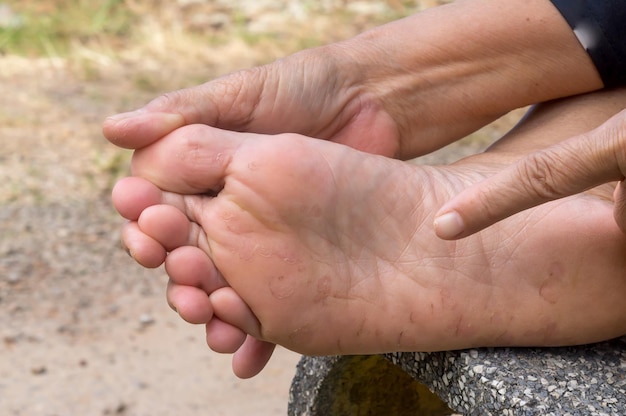In this detailed outdoor image, a person's right foot is prominently displayed, resting on a dark gray, granite-like surface with white and gray flecks. The foot, relatively clean but with some faint markings and visible blue veins, spans horizontally from right to left near the center of the picture. The person's right hand is grasping the top of the foot, pressing down on the smaller toes with the thumb, while the left hand uses the index finger to point towards the bottom of the foot. The hands and arms extend from the upper right corner of the image. A dark blue sleeve is partially visible on the right wrist. The background features a mix of light brown soil, gravel, and patches of green grass, providing a natural setting for the scene. The person seems to be highlighting something specific on the sole of their foot amidst this earthy outdoor environment.